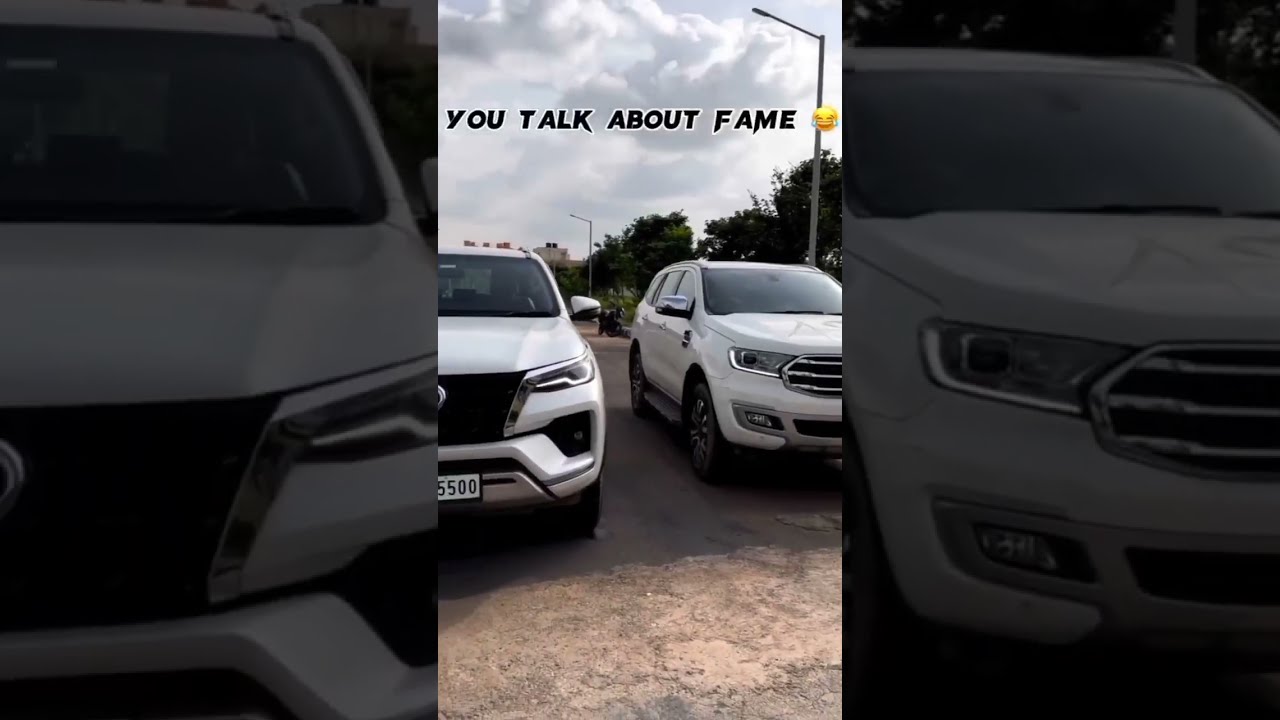The image is a rectangular outdoor photograph of two white SUVs, a Ford and a Toyota, positioned side by side facing the viewer, with a small gap between them and the right vehicle slightly set back. The SUVs are parked on a worn asphalt road that could use resurfacing, surrounded by a concrete ground. In the background, dense grey-black clouds fill the sky, with a hint of sunlight peeking through, possibly suggesting impending rain. The background also features trees, bushes, and two unlit street lamps. Overlaying this scene, a central brighter image presents the same view but from a slightly farther back perspective and is framed by a grayed-out larger version of itself, creating a border. The caption "You Talk About Fame," accompanied by a crying-laughing emoji, is prominently displayed across the top of the central image. Additionally, there is a bumper sticker visible on one of the vehicles, and the number "550" is seen on the left SUV.